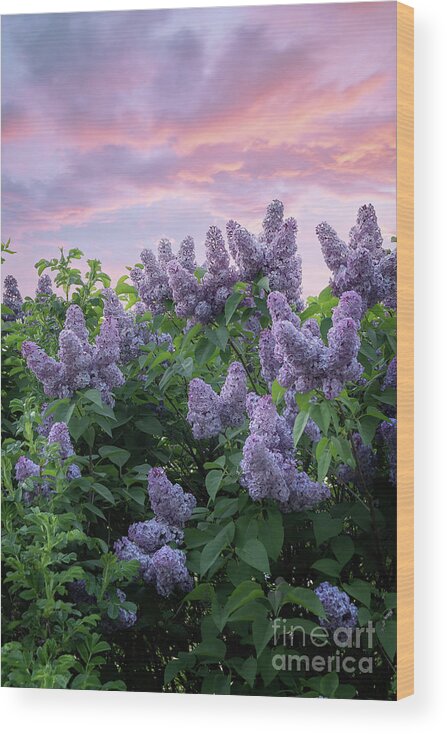This artwork canvas portrays a vibrant outdoor nature scene during sunrise or sunset, organized as a vertical, portrait-oriented image. The canvas features a field of lavender flowers in full bloom, filling the bottom two-thirds of the frame. These lilac-colored flowers, which are cone-shaped and composed of very tiny purple leaves, stand upright and are surrounded by clusters of bright green leaves. Each cone measures approximately three to four inches in length, with two to four cones per cluster. The upper third of the canvas displays a serene skyscape in hues of blue, pink, purple, and orange, suggesting the tranquil time of dawn or dusk. The right-hand side of the long rectangular canvas is bordered by a light wooden edge. A watermark reading "Fine Art America" appears in faint white letters in the bottom right-hand corner of the image. The image's slight angle enhances the perspective, emphasizing both the edge of the canvas and the natural beauty of the lavender field.